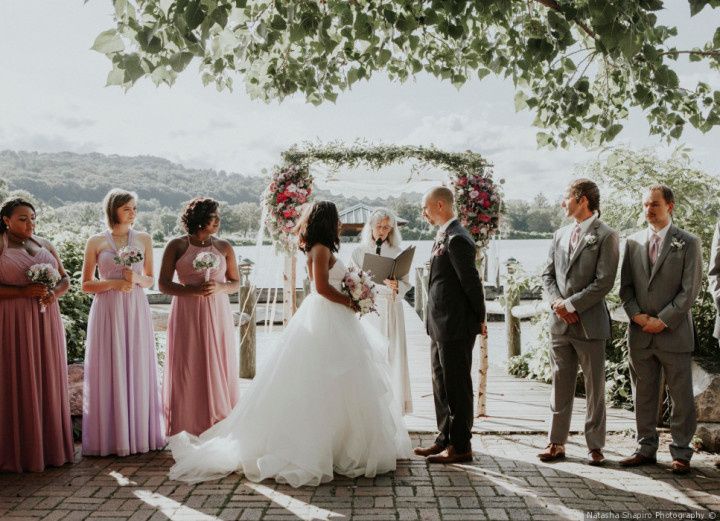In this vibrant outdoor wedding scene, the bride and groom stand at the altar in front of an officiant under a decorated arch adorned with white flowers and greenery. Above them hangs a tree branch embellished with more white flowers. The backdrop is a picturesque view of mountains and serene water, adding a touch of natural beauty to the ceremony. 

The bride, an African-American woman, exudes elegance in a form-fitting white dress with fluffy ruffles cascading down. She holds a bouquet of pink and white flowers. The groom, a white man, looks sharp in a classic black tux with a white shirt, his hands clasped behind his back.

To the left of the couple, three bridesmaids—dressed in varying shades of pink and purple—each clutch small bouquets of white flowers. Among them are two African-American women and one white woman. On the right stand two groomsmen in gray tuxedos, both white, complementing the groom's attire.

An older white woman with white hair, the officiant, conducts the ceremony with a book and microphone in hand. The cobblestone-like tiles beneath their feet lend a rustic charm to the setting, making it a quintessential moment worthy of a wedding magazine or cherished family album.